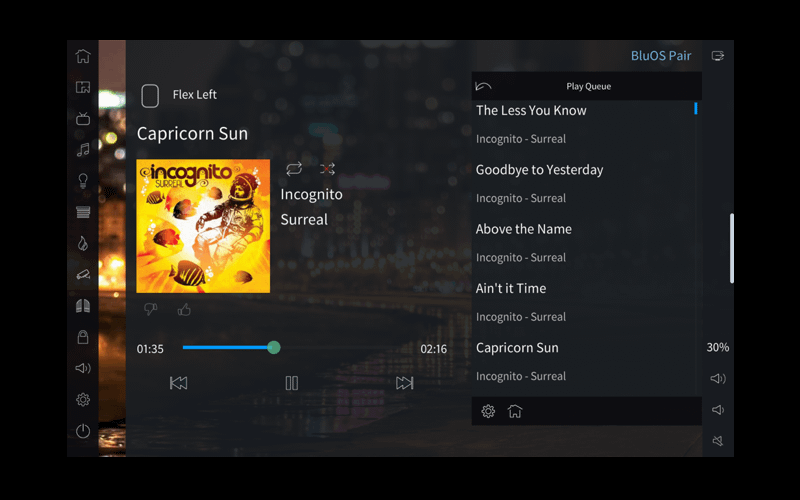The image features a black border encompassing a digital interface. Towards the middle left of the screen, there's an album cover predominantly yellow in color, depicting an imaginative scene with several fish swimming around and an astronaut floating by. The album cover has "Incognito Surreal" prominently displayed on it, with "Flex Left Capricorn Sun" written above.

To the right side of the album cover, "Incognito Surreal" is again written, and beneath it lies a play menu. The play bar within the menu is paused at 1:35, indicating that there are 2 minutes and 16 seconds remaining in the track. Above this menu, the words "Play Cue" appear, while below it, the tracklist is displayed with the current, past, and next songs.

The tracklist includes:
1. "The Less You Know" by Incognito Surreal.
2. "Goodbye to Yesterday" by Incognito Surreal.
3. "Ain't It Time" by Incognito Surreal.

The album title "Capricorn Sun" is shown at the bottom of the tracklist, reiterating the thematic linkage between the album, band, and song titles.